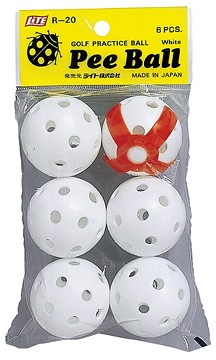The image depicts a package of six white practice golf balls arranged in a 2x3 grid (two wide and three deep) against a medium gray background. The top right ball is distinctively marked with a red circle and four red stripes extending from its center. These balls, which resemble wiffle balls with their plastic construction and perforations, are labeled as "P-Ball" and are described as "Golf Practice Ball" on the packaging. The tag at the top of the package features a yellow background with a black ladybug motif and additional labeling in Japanese, indicating the product is made in Japan. The tag also includes the text "six pieces," "light," and "R20." The combination of detailed packaging and distinctive ball design highlights the functional and playful elements of these practice golf balls.